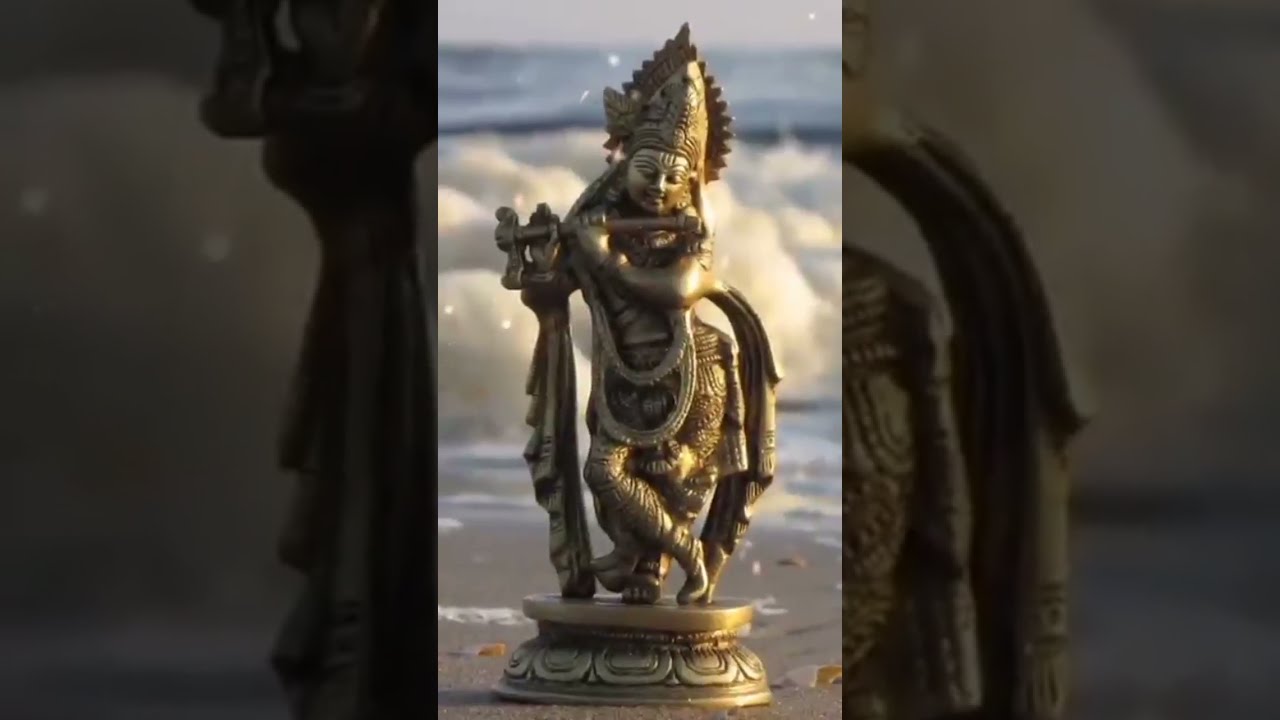In this photograph, we see a detailed bronze Krishna statuette situated on a beige sandy beach with white, crashing ocean waves in the background. The statuette, which stands on a round, carved pedestal, depicts Krishna playing a flute held close to his mouth. He is adorned in elaborate attire, featuring an extensive headdress or helmet with a triangular peak, long pants, and long-sleeved robes that drape gracefully. The figure's legs are elegantly crossed in front of him, and he wears two long strands of thick gold beads that hang past his hips. The intricate carvings on the headdress, pants, and pedestal add to the ornate appearance of the statuette. The scene captures a serene moment with the dynamic ocean waves behind, highlighting the contrast between the stillness of the statue and the movement of the sea. The surrounding sand, embedded with small rocks, and the hint of a border created by grayed-out portions of the image, encapsulate the peaceful yet majestic presence of Krishna on the beach.